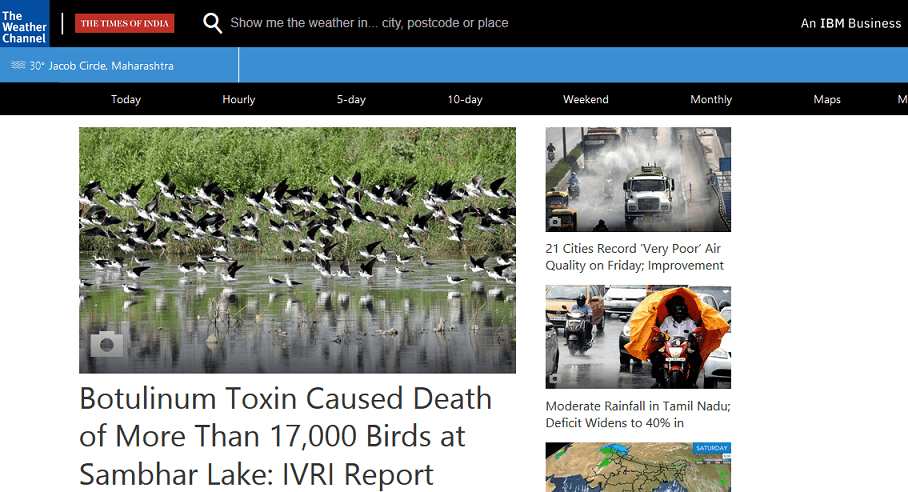A detailed screenshot of a Weather Channel application displayed on a computer screen. At the top, the Weather Channel logo is present, alongside a clickable button labeled "The Times of India". Directly below, there is a search bar with the prompt "Show me the weather in" where users can input a city, postal code, or place. The screen indicates that the Weather Channel is an IBM Business. Beneath the header, a blue bar displays the temperature as 30 degrees in Jacob's Circle, Maharashtra.

A black navigation bar below the temperature spans horizontally with options including Today, Hourly, Five Day, Ten Day, Weekend, Monthly, and Maps. This bar allows users to explore different weather forecasts and maps.

Below the navigation bar, an image of numerous waterfowl in flight is shown, accompanied by a distressing news headline: “Botulinum toxin causes death of more than 17,000 birds at Sambar Lake, IVRI report.” Down the right side of the screen, a series of additional articles are listed: "21 cities record very poor air quality on Friday," "Record improvement, moderate rainfall in Tamil," and "Deficit widens to 40%." A partial map is also visible, though its details are not fully displayed.